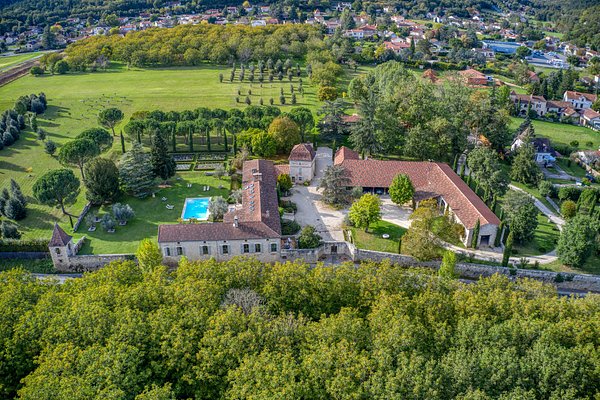This is a vibrant aerial photograph taken on a pleasant day, capturing a large property surrounded by lush greenery. In the foreground, the entire bottom of the image is densely covered with leafy green trees, creating a sense of seclusion and privacy. The main focus in the center of the image is two large L-shaped buildings with white walls and brown roofs. The left building features a small church-like steeple. Both buildings are situated on a well-manicured, expansive green lawn, with a distinctive, eye-catching swimming pool nestled between them. The property is clearly demarcated with a stone fence and dense stands of various types of trees, including some pines, adding to its seclusion. In the background, the scene stretches out to reveal a multitude of smaller white buildings with brown roofs extending across the top of the image, interspersed with more stands of trees. This area leads into a distant cityscape with numerous buildings and roads, providing an impressive contrast between the serene, private mansion in the foreground and the bustling city beyond.